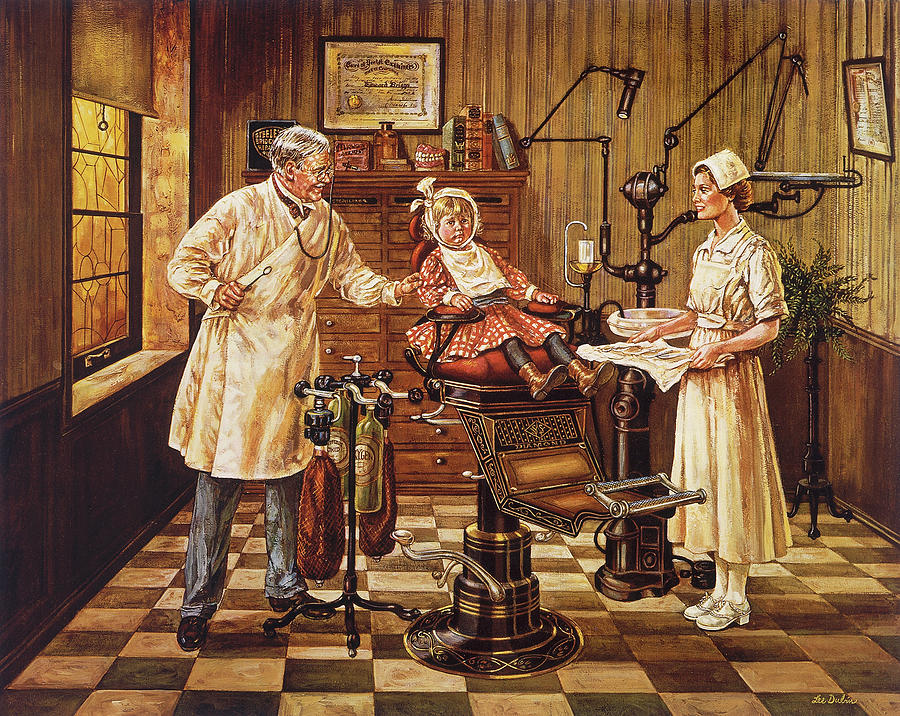The image is a detailed painting of a young girl, likely around four years old, sitting in an elevated dentist's chair reminiscent of an old-fashioned barber's chair, possibly from the early to mid-20th century. The girl, who may appear older or perhaps has a mature face suggestive of dwarfism, is dressed in a red and white checkered dress, black stockings, and brown shoes. She has a cloth bandage wrapped over her head, possibly to support an ice pack for a swollen jaw, and a bib around her neck. Her legs dangle off the edge of the chair, which is supported by a visible pole extending downward.

On either side of the girl are two adults: to her left stands an older man, the dentist, wearing a white lab coat and gray pants, and to her right is a nurse in a long white dress holding a tray of dental tools covered with a white cloth. The room has brown-tinted walls and features a window on the left. The floor is a distinctive black and white checkerboard tile. Behind the girl, there's a large wooden chest of drawers and a gas tank, possibly containing nitrous oxide, suggestive of the era's dental equipment. A plant is placed near the right side of the painting. The room exudes a vintage atmosphere, enhanced by the brownish hue of the walls and the furniture. The artwork is signed by the artist, though the signature is too small to read clearly.